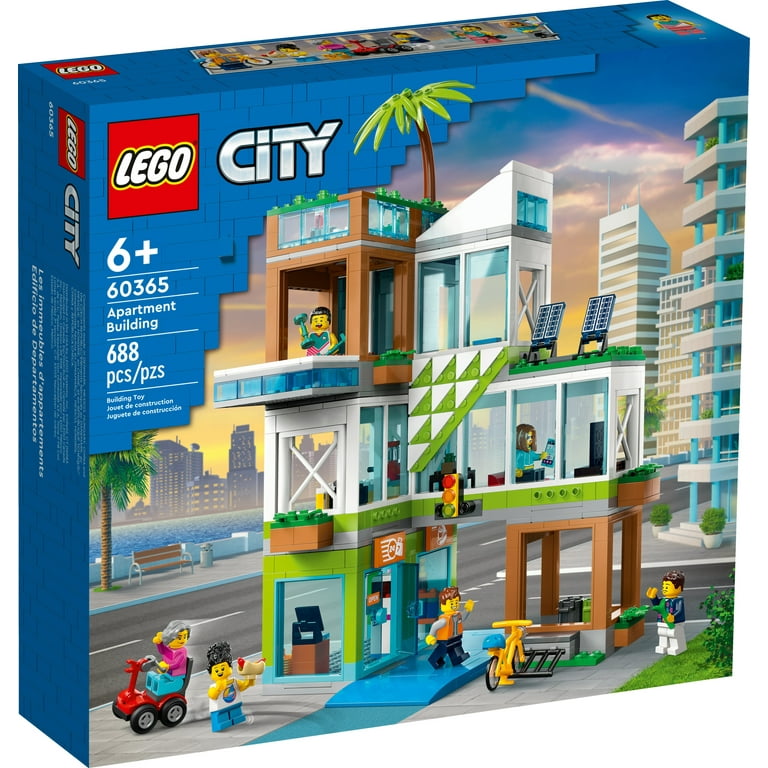This is an image of a LEGO City set. Prominently displayed at the top left is the iconic LEGO brand symbol, a red background square with the LEGO text outlined in yellow. Adjacent to it is the "City" logo in italicized blue text. The set is identified for ages 6 and up, with the model number 60365, aptly named the “Apartment Building,” comprising 688 pieces. This is a product image with no distinguishable background, focusing solely on the package. The box, displayed on its thin side and slightly tilted to the right, features a vibrant blue background. The design on the box illustrates a modern, eco-friendly apartment building. The structure includes a balcony at the top where a minifigure is visible, a rooftop equipped with solar panels, and another recognizable silhouette of a palm tree. At the ground level, there's a cozy cafe patio, with a parked yellow bicycle visible beside it. Several LEGO minifigures are depicted engaging with the scene, including one riding a scooter and a couple waving to each other. Additional elements such as a palm tree and varied apartment interiors detail the vibrant, bustling miniature community. The packaging also includes repeated texts in multiple languages outlining the number of pieces and the nature of the building toy.